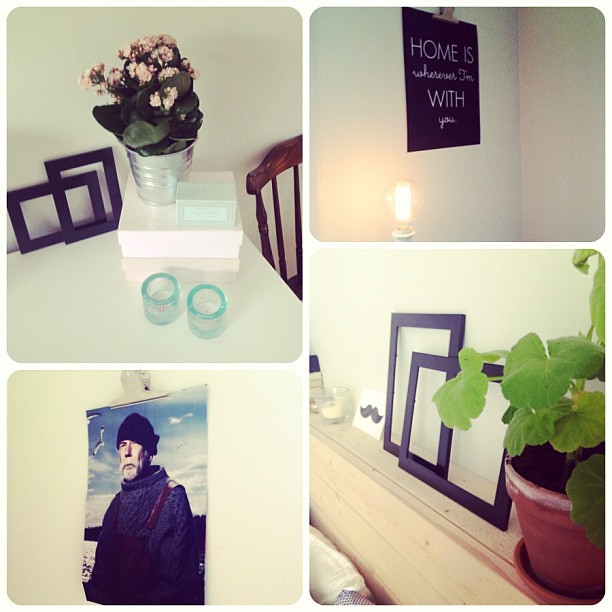This composite image consists of four individual photographs arranged in a two-by-two grid. 

**Top Left:** A rounded rectangle displays a white table situated in front of a white wall. On the table, near its edge, is a box with a metal bucket filled with flowers placed on top. In front of the box, there are two glass candle holders without candles. Behind the table and to the left, two black picture frames are visible, while a wooden chair stands to the right.

**Bottom Left:** Within a rounded square, there is a poster of an elderly man in a blue sweater and stocking cap. The man, with a white beard and mustache, is depicted against a backdrop of the sky and birds, making it seem like he is standing near a lake or open landscape. He also appears to be wearing overalls over his sweater.

**Top Right:** A rounded square contains a décor item hanging on a white wall. The hanging, featuring a maroon background with white text, reads "Home is wherever I'm with you." Just below this hanging, a bright bulb without a lampshade is visible.

**Bottom Right:** The rounded rectangle here shows a wooden shelf mounted diagonally from the middle left to the bottom right of the image. This shelf holds three picture frames in the middle, a potted plant on the bottom right, and other indistinct items on the upper left. The shelf is backed by a white wall and appears to be mounted above an indeterminate fabric-covered object in the bottom left corner, possibly a couch.